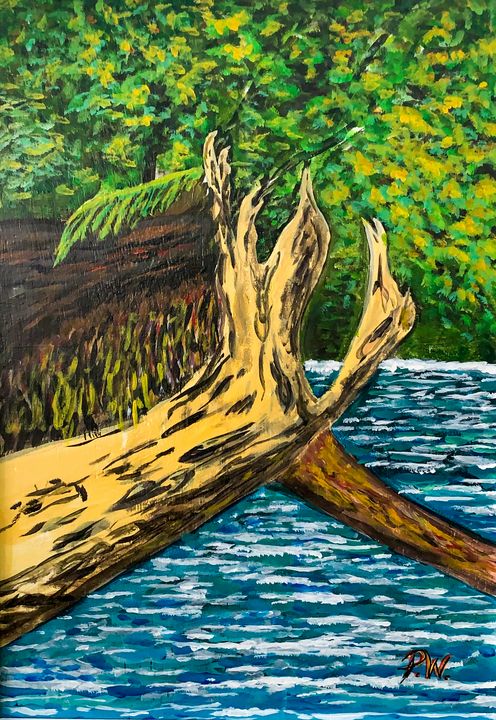This vertical acrylic painting depicts a serene natural scene with a focus on a river or creek running through the foreground. Dominating the composition is a fallen log, brown in color with a protruding branch on the right, which appears to serve as a natural bridge over the blue and white water. The river itself shows motion through its fluid, light brushstrokes. Just beyond the log, a large brown rock can be seen, further adding to the rustic ambiance. The background showcases a vibrant forest with a blend of deep yellow, light green, and dark green foliage, created with thick, blotchy brushstrokes that suggest either an impressionistic influence or an amateur level of artistic technique. Despite its lack of refined detail and stylistic subtlety, the painting captures the essence of a peaceful woodland scene. In the lower right-hand corner, the painting is signed with red initials, which appear to be RW.